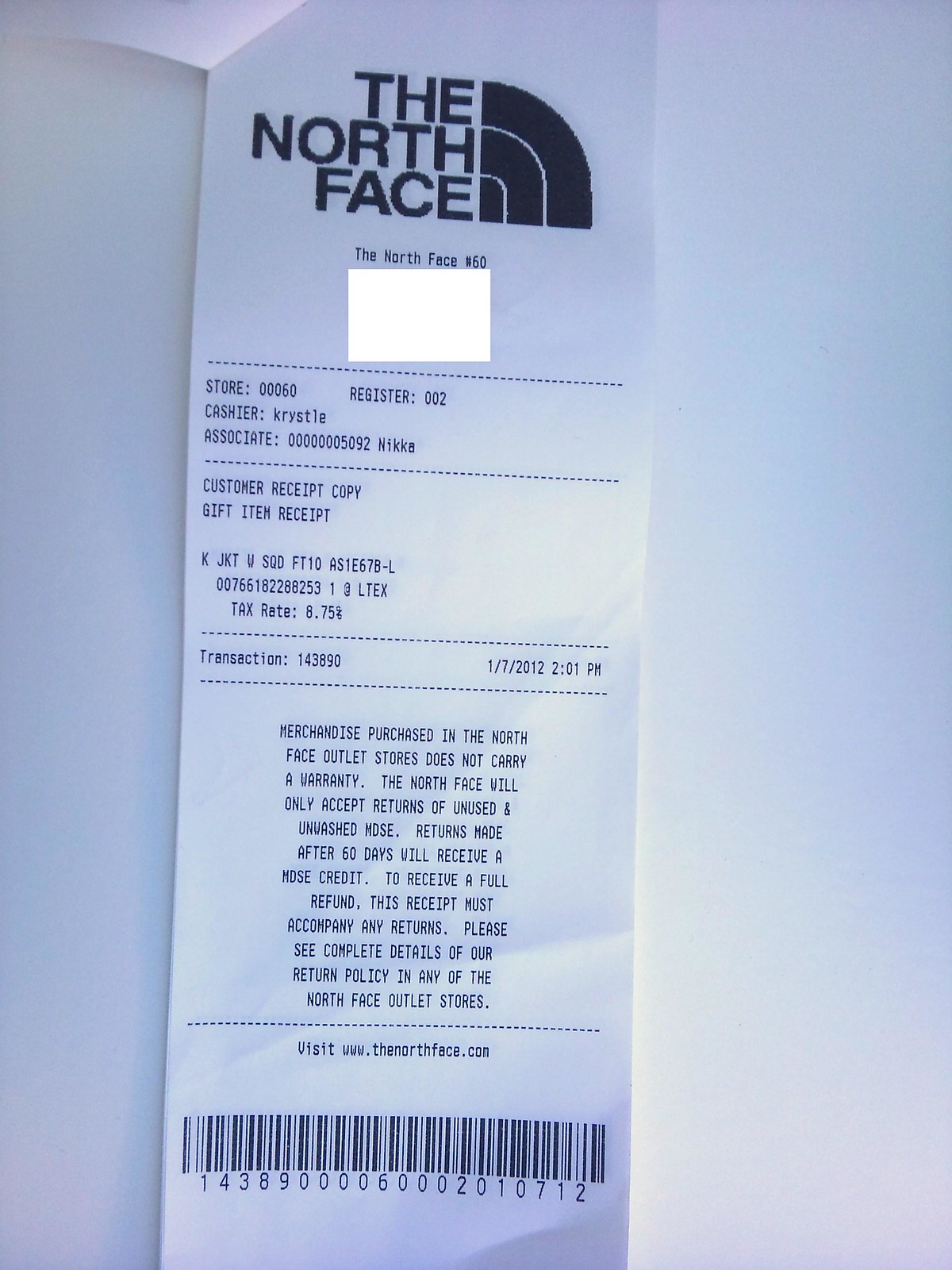The image features a North Face receipt set against a grayish-blue background that fades to white in the center. The receipt itself is predominantly grayish-white with black lettering. At the top, it prominently displays "The North Face" along with their rainbow-style logo. Details include store number 00060, register 002, and cashier Krystle (spelled K-R-Y-S-T-L-E), associate number 1592. The receipt mentions a gift item with the identifier KJKTWSQDF10AS1E67B-L and indicates a tax rate of 8.75%. The transaction number is 143890172012, timestamped at 2:01 PM on January 7, 2012. There's a white box on the receipt likely covering personal information. It includes a note that merchandise purchased from North Face outlet stores does not carry a warranty, and that returns of unused and unwashed items are accepted within 60 days with a full refund given only if the receipt accompanies the return. Any returns made after 60 days receive a merchandise credit. The receipt ends with a barcode and the website www.thenorthface.com for further details on the return policy.